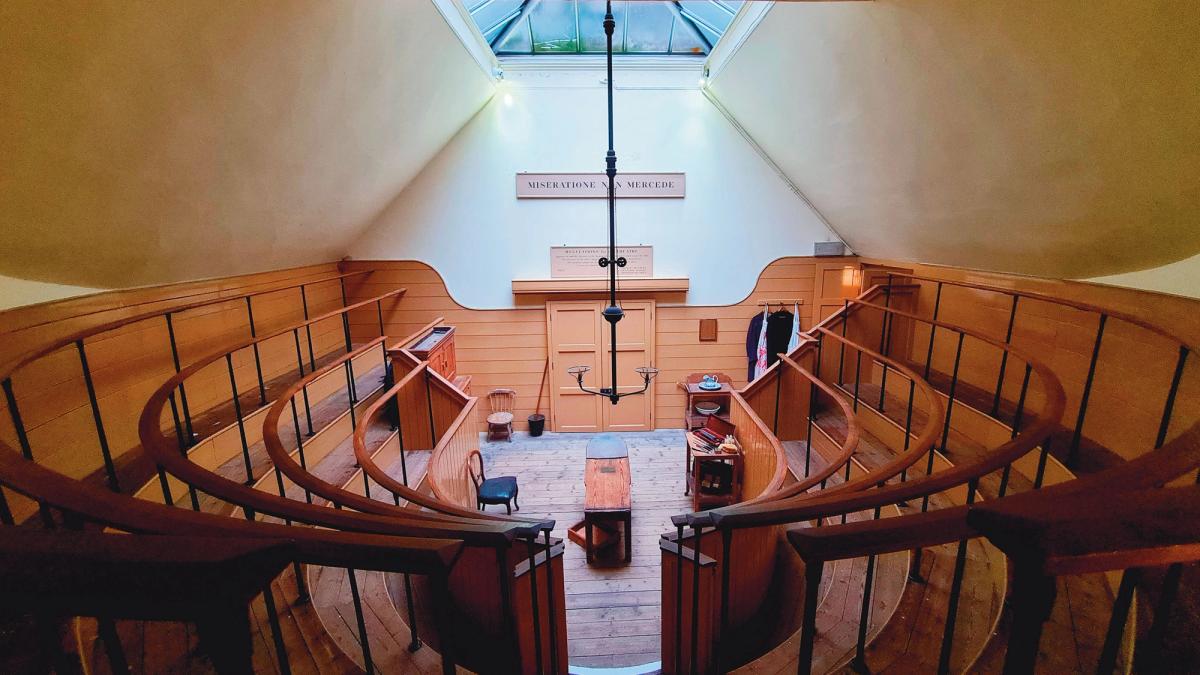This photograph captures an indoor scene inside a distinct auditorium-like room with features suggesting it may be located in a foreign country. The focal point is a slanted white ceiling, partially made of large slabs and incorporating a skylight that allows natural light to flood the room. Prominently hanging from the ceiling is a long metal pole adorned with several lights, positioned above a central wooden table.

The space is organized with four curved rows of seating that descend towards the bottom, enclosing a floor of polished brown wood. Furniture on this floor includes a couple of wooden tables, a dresser, a plain wooden chair, and another chair with a blue seat. The room has risers bordered by banisters, and a stairway leads down to the middle floor, suggesting it's designed for large gatherings or lectures.

At the back of the room, the medium brown wall features multiple signs, with partially visible words reading "MISERATIONE" and "MERCEDE." Above these, additional signs with more text are present but obscured. There are double doors towards the back. The photo is in full color and horizontally rectangular. No people, watermarks, or set borders are visible, allowing the architectural and design details to stand out prominently.